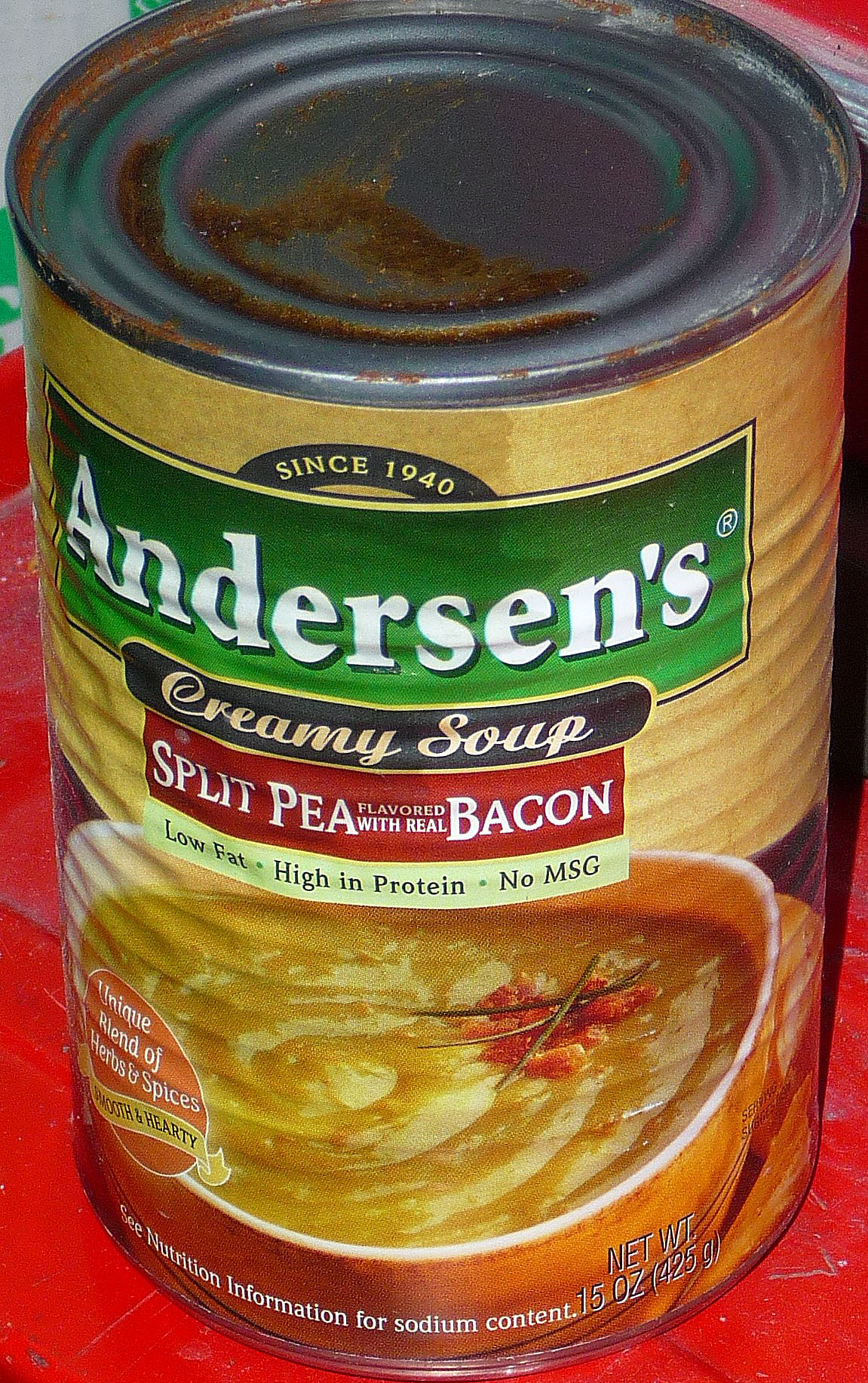This is a close-up photograph of a can of Anderson's Creamy Soup, Split Pea flavor with real bacon, taken indoors under kitchen lighting. The can, which appears old and is labeled with the brand's establishment date "since 1940," stands on a red surface. The top of the can is notably rusty, especially around the edges and extending towards the center. The label is predominantly cream-colored with a green rectangle featuring the brand name "Anderson's." Below, it states "creamy soup split pea with real bacon," followed by icons highlighting "low fat, high in protein, no MSG." There is an illustration of the soup in a bowl, showing bacon bits and three herb sticks. An orange circle on the label emphasizes a "unique blend of herbs and spices" with a banner reading "smooth and hearty." Nutritional information is indicated, advising to "see nutrition information for sodium content." The net weight of the can is specified as 15 ounces (425 grams).